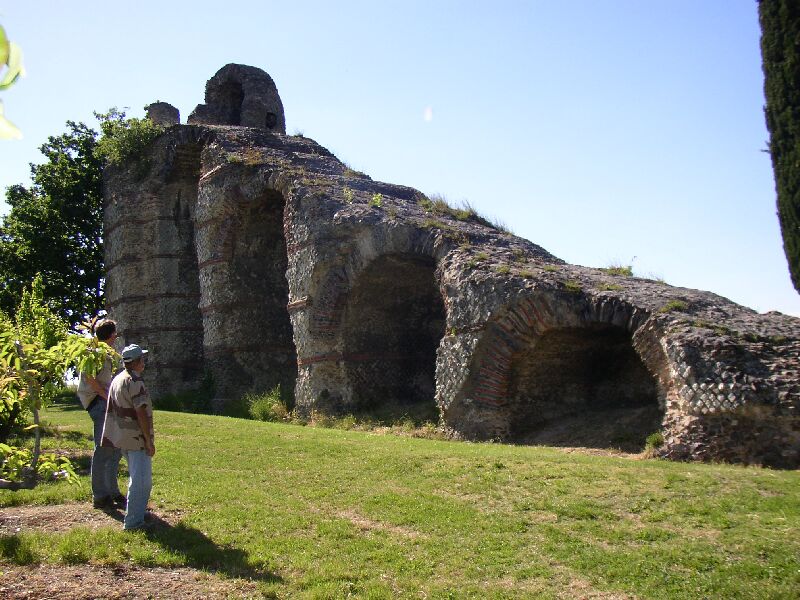The image captures an ancient stone structure, weathered and partly destroyed, sloping upward from right to left. The structure, likely from a bygone era, features multiple entrances reminiscent of cave entryways; three of which are distinctly visible with varying sizes—the smallest being circular on the right, a taller one in the middle, and the largest one on the left. The formation appears to have once been a stairway and exhibits patches of grass on its surface, indicating its age and natural integration into the landscape.

In the foreground, two men, both in blue jeans and short-sleeved shirts, are standing on grass, with one area appearing brown and dirt-like. They intently observe the structure, the man on the left in a brown shirt and the one on the right wearing a hat and a brown and black shirt. Surrounding the scene is a vivid outdoor setting bathed in the middle of the day’s sunlight, showcasing a bright blue sky. To the left of the structure, there is a mix of large and small trees, along with a green bush partly visible behind them. The composition of the scene combines natural and historical elements, providing a glimpse into a site of archaeological interest.